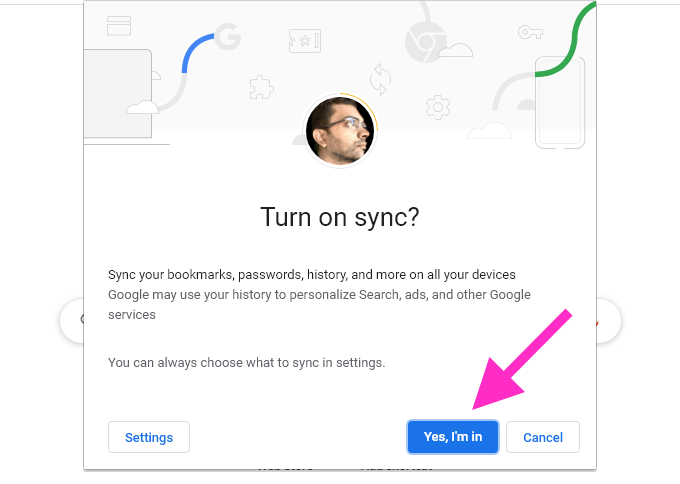This image is a screenshot of a pop-up notification on a website or application. The background is predominantly white, featuring a thin light gray line running across the top. At the bottom of the pop-up, there are two white circles casting light gray shadows.

The main content of the pop-up also has a white background. At the top, there is a light gray header displaying various cartoonish icons outlined in dark gray. On the left side of the header, there's an icon of a computer with an "S" shape coming out of it, transitioning from a blue top curve into a gray "G" among other icons.

Central to the pop-up, overlapping both the light gray header and the white main body, is a round profile picture icon surrounded by a thin light gray circle, except for the top right quadrant which is highlighted in orange.

Below the profile picture icon, large black text reads, "Turn on sync." This is followed by a smaller paragraph in black text spread across three lines:

"Sync your bookmarks, passwords, history, and more on all your devices. Google may use your history to personalize search, ads, and other Google services."

A couple of line breaks down, another sentence reads:

"You can always choose what to sync in settings."

In the bottom left corner of the pop-up, a white rectangular button with rounded corners, a thin gray outline, and blue text in the middle reads, "Settings." 

Similarly designed, a button on the bottom right reads, "Cancel," in blue text. Next to it, a blue button with a thin light blue outline and white text in the middle reads, "Yes, I'm in." Notably, a pink arrow points to this blue button from the top right, suggesting it is the preferred choice.